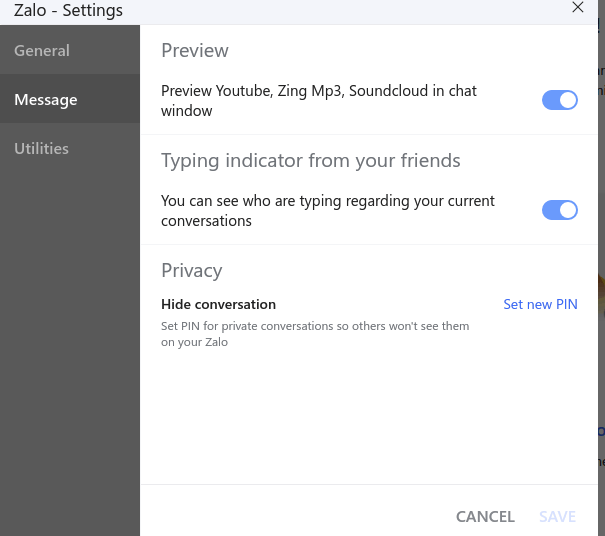The image depicts the settings page of a chat application with various customization and privacy options. The interface shows a series of sections labeled 'Settings,' 'General,' 'Message Utilities,' 'Preview,' 'Preview YouTube,' 'Zing MP3,' and 'SoundCloud.' Each section offers different functionalities. 

In the 'General' and 'Message Utilities' areas, users can see who is typing in their current conversations, thanks to the 'Typing Indicator for your friends' feature. The 'Privacy' section includes options to hide conversations and set a PIN for private chats to ensure they remain unseen by others.

The 'Preview' settings provide light grey and dark grey themes for the chat window, and include preview options for integrating YouTube, Zing MP3, and SoundCloud content directly into chats. Additionally, there's a blue oval toggle switch with a white circle positioned to the right, indicating activation.

Throughout the interface, different elements are color-coded, such as the grey 'Privacy' option, black 'Hide Conversation' option, and the 'Set New PIN' feature, which includes functionality to either set a new PIN or cancel the action.

Lastly, the background of the page appears to be greyed out, likely highlighting the active settings interface in the foreground.